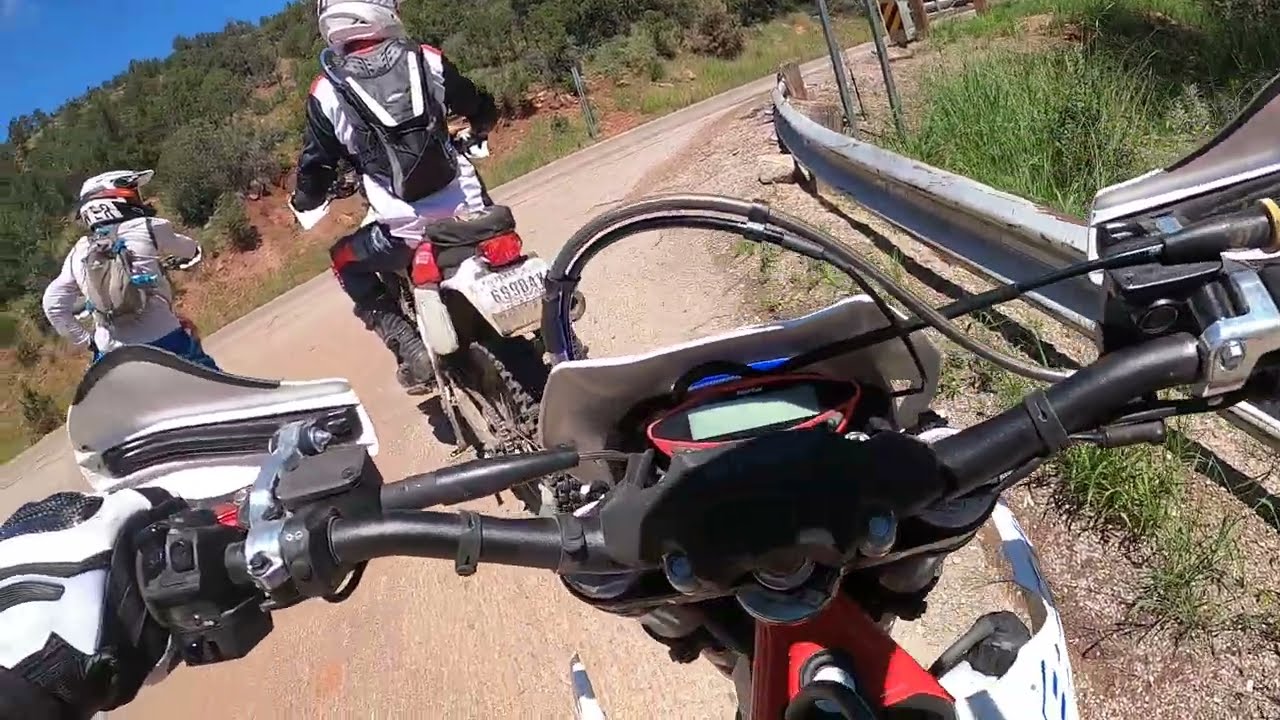In this picturesque rural setting, three individuals are captured riding dirt bikes, fully geared for off-road travel. The image offers a sweeping view of a gravel road lined with a metal guardrail on the right-hand side, curving gently from the center to the top right of the frame. The photograph is taken from behind the foremost rider, whose black dirt bike, accentuated with red details and a speedometer, occupies the lower half of the image. The rider's hands, clad in black and white gloves, grip the handlebars, angling the perspective at about 30 degrees from bottom left to top right.

Ahead, in the upper left third of the picture, another rider on a dirt bike is visible, accompanied by a third rider to the far left. Both riders are dressed in white and black protective gear, equipped with helmets and CamelBak backpacks, suggesting they are prepared for a rugged journey. The riders appear to be navigating a turn, their attire featuring white jackets, black and white pants, and shin guards standing out against the neutral tones of the road and guardrail.

Surrounding the scene, the landscape is dotted with low bushes and grasses, with rolling hills visible in the distance to the left. The sky is a vibrant blue, occupying the upper portion of the frame and contrasting with the greenery below. Despite the arid environment, this outdoor snapshot beautifully captures the thrill of a dirt biking adventure amidst the rugged, open countryside.